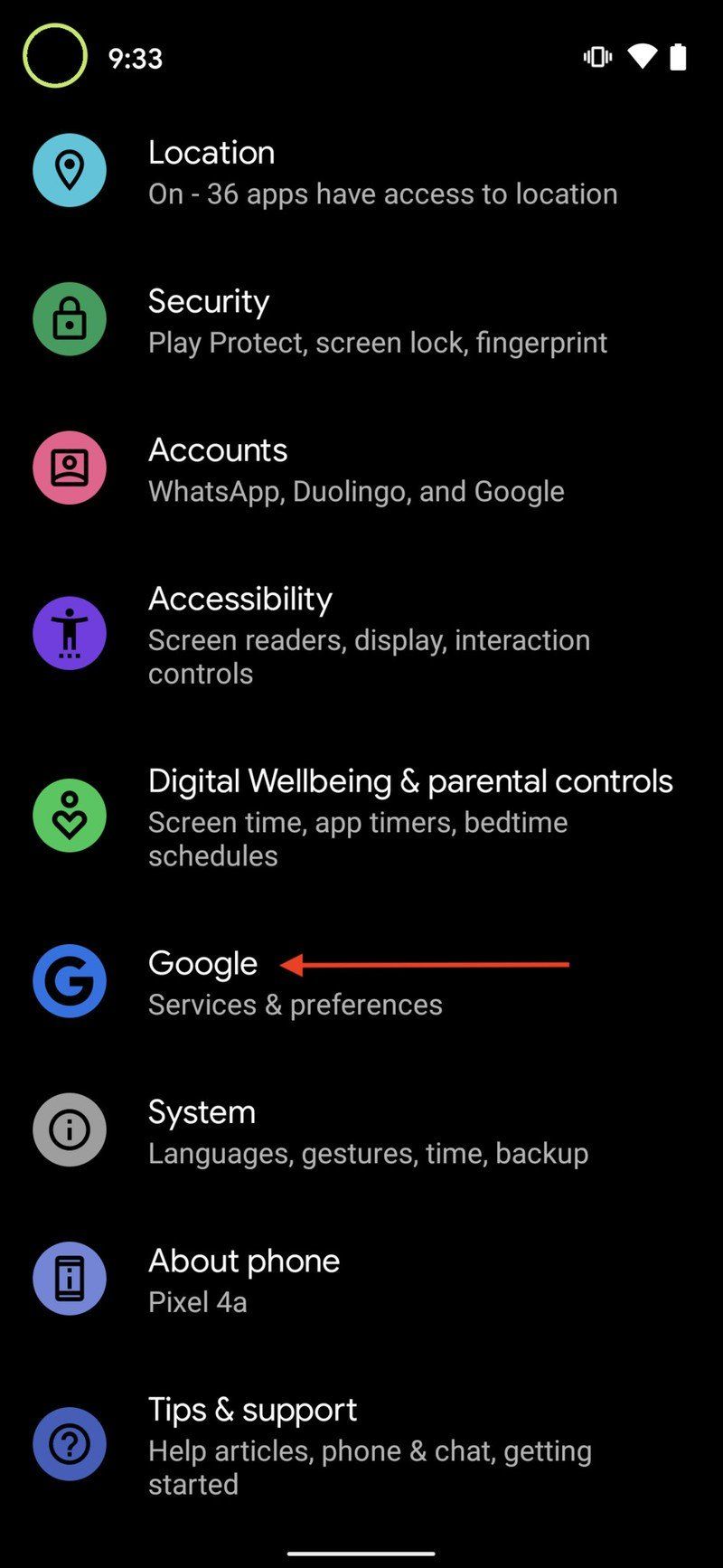In the provided image, a smartphone screenshot is displayed featuring a variety of interface details. The top right corner showcases a fully charged battery icon in white color, left of which is a complete Wi-Fi signal strength icon, and next to this is a phone vibration icon. On the top left, a small light green circle is present, followed by the time "9:33".

Beneath these status icons is an organized list of settings categories, each with succinct descriptions:
- **Location:** Indicates "On" status and reveals that 36 apps have access to location services.
- **Security:** Lists elements such as "Play Protect," "Screen locked," and "Fingerprint."
- **WhatsApp, Duolingo, Google:** A category grouping these apps.
- **Accessibility:** Includes features such as "Screen readers," "Display," and "Interaction controls."
- **Digital Wellbeing and Parental Controls:** Describes features like "Screen time," "App timers," and "Bedtime schedules."
- **Google:** This category is highlighted with a red arrow pointing at it.
- **System**
- **About phone**
- **Tips and support**

Each category is stacked below the previous, creating a comprehensive overview of the phone's settings at a glance.